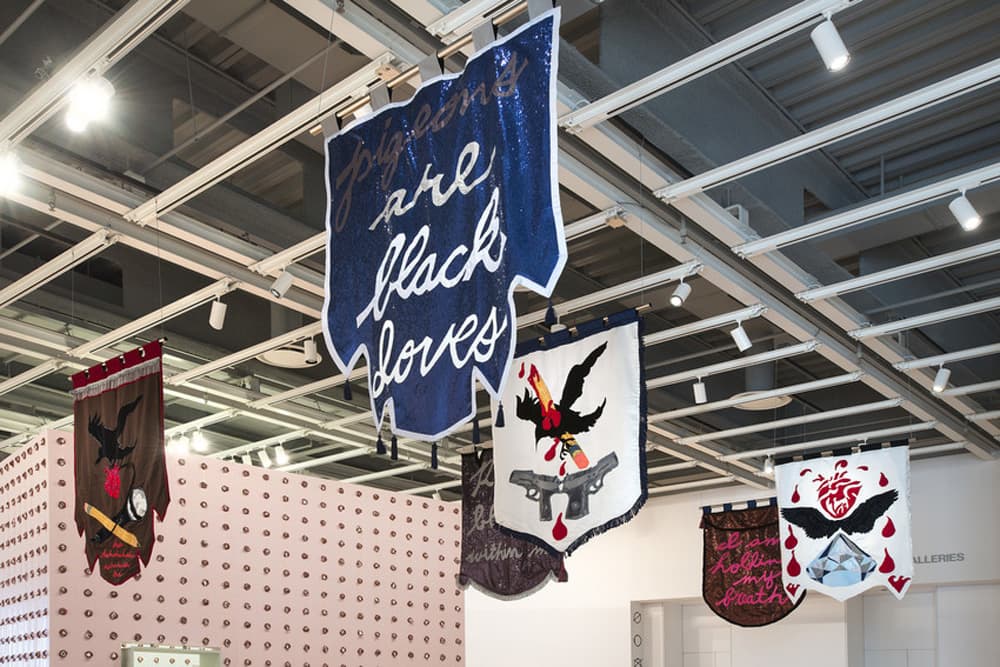This vibrant color photograph captures an upward view of a greyish roof framed by several silvery metallic beams arranged in a rectangular pattern. Hanging from the roof are a variety of flags and mascots, adding to the lively atmosphere.

At the bottom of the image, a pink wall with circular cutouts is visible. To the backdrop, a white wall dominates, with a grey wall situated in the left-hand corner. On the left side, a greyish-brown flag featuring a central "X" design is prominently displayed. Below the "X," there are symbolic elements including a red ball, what appears to be a sword or possibly a bat, and a white ball.

Centered in the image is a blue flag with a white outline, inscribed with black text. At the bottom of this flag, motifs resembling either gloves or the word "loves" can be observed. Behind this flag, a white flag is depicted featuring a black eagle in flight, clutching two guns in its talons.

Further back, a series of flags add to the array: a brown flag with white writing, another brown flag with pink writing, and finally a white flag located in the far left-hand corner. This latter flag showcases an intricate emblem in the center, featuring two black wings bordered by red feathers, with a diamond shape at the bottom and an unidentifiable red object at the top, adding an air of mystery to the scene.